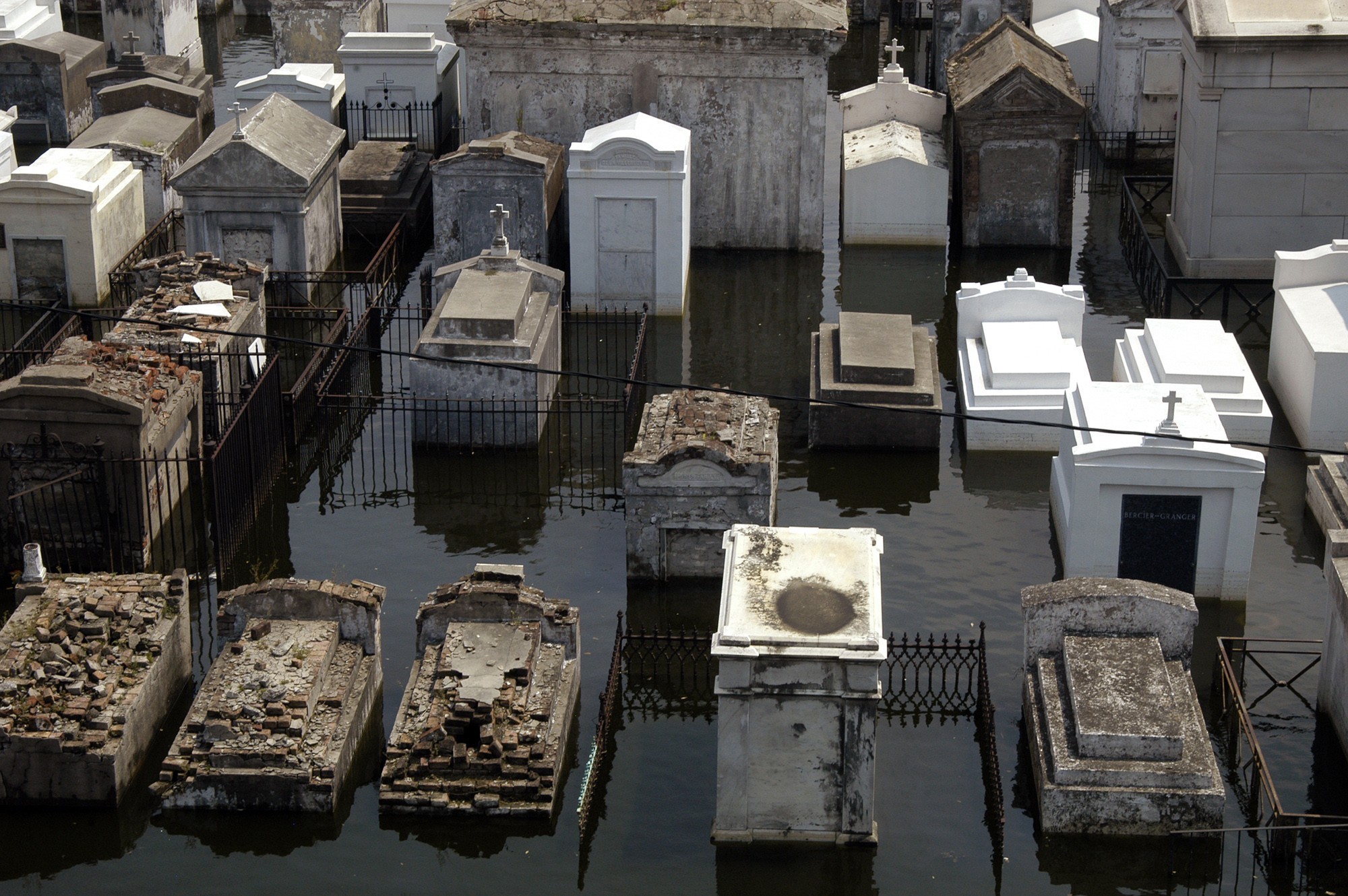This photograph, taken from an overhead perspective, captures a flooded cemetery reminiscent of those in New Orleans, where tombs are constructed above ground due to frequent flooding. The image, in landscape layout, prominently displays dark, almost black, muddy water partially submerging approximately twenty varied structures. These structures, appearing as small mausoleums or vaults, differ widely in condition and color, ranging from deteriorated browns and grays to pristine whites. Several newer, clean white tombs bear crosses atop, while older ones exhibit signs of decay with chipped bricks and stones. There are wrought iron fences surrounding some, adding an antique feel, and a visible wire, likely a telephone line, runs through the center. Stone walls with gray streaks frame the background, and scattered rubble from partially destroyed tombs is noticeable at the bottom. No people or text are present in the image.